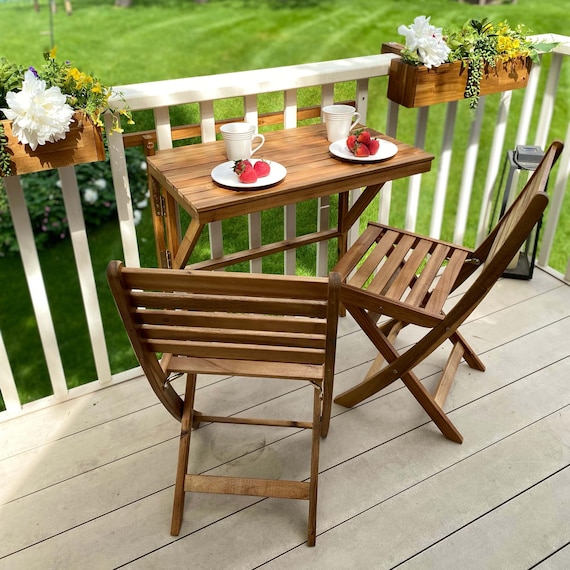The image depicts a meticulously maintained porch area, likely a deck, featuring a quaint and inviting setup. At the center is a small wooden table, accompanied by two slatted wooden chairs placed catty-corner to each other. Each chair is positioned beside the table that holds two plates of strawberries and two white coffee cups, neatly arranged in front of and behind the plates. The deck and its railings are made of pristine white wood, adding to the clean and serene ambiance of the space. On the right side of the porch railings, two planters brimming with white, yellow, and green foliage hang gracefully. A similar planter can be seen to the left, enhancing the uniformity and aesthetic of the decor. From this elevated viewpoint, a beautifully manicured lawn stretches out, showcasing clear tracks from recent mowing. In the background, a variety of bushes and possibly some trees add depth and natural beauty to the serene porch setting.